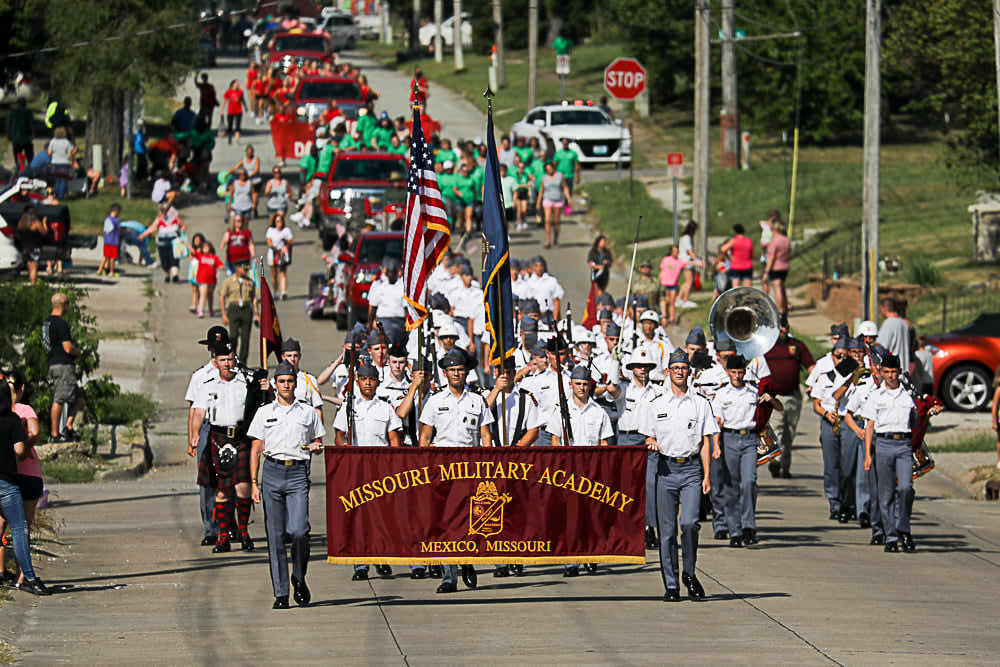This color photograph captures a vibrant daytime parade featuring the Missouri Military Academy in Mexico, Missouri. Leading the procession are two soldiers carrying a prominent maroon banner with gold writing that reads "Missouri Military Academy, Mexico, Missouri." The banner's center showcases the academy’s shield logo, which features a diagonal rod, all in gold. The banner is adorned with gold frills at the bottom and stands out against its red background. 

The front-line soldiers are dressed in uniforms consisting of white shirts, slate-colored pants, and black dress shoes, with one notable exception: a man in a red and black checkered kilt paired with red and black socks, who carries bagpipes. Among the soldiers, some are holding rifles on their right side, and there are also flags being carried, including the American flag and another slate-colored flag with an indiscernible design.

Behind this leading formation is a diverse array of participants, including a marching band with at least one musician playing a silver tuba. The parade stretches along the street, featuring various individuals and groups. Notable among them are a group wearing green shirts and another group dressed in red shirts, as well as floats and numerous vehicles, some of which have clusters of participants surrounding them. 

The scene is further animated by a police car with flashing lights parked on the left side of the road, indicating the parade route. The parade attracts several onlookers who line both sides of the street, enjoying the event under the green canopy of trees.